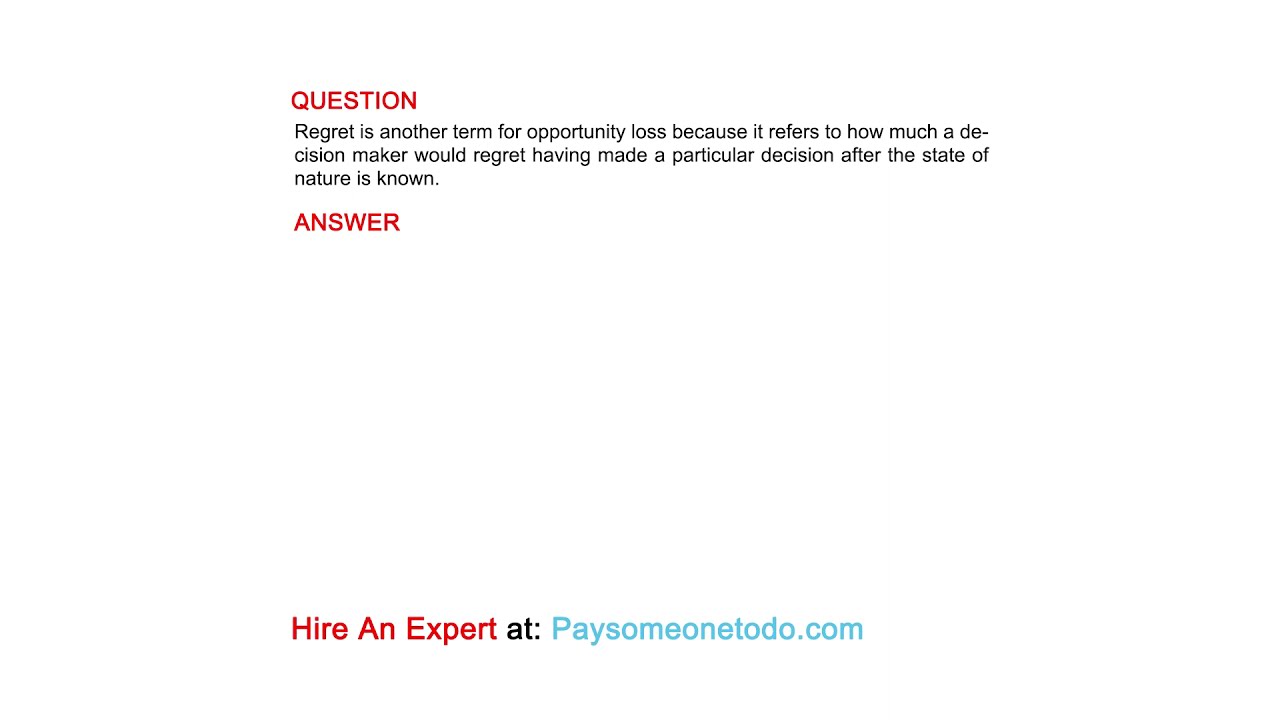The image is a text-based ad with a white background. At the top, "QUESTION" is written in red font, followed by black text that reads: "Regret is another term for opportunity loss because it refers to how much a decision maker would regret having made a particular decision after the state of nature is known." Below this explanation, in larger red font, is the word "ANSWER," which is followed by a large white space, indicating that the answer has been redacted or is missing. At the very bottom of the image, there is a call to action: "Hire an expert" in red font, followed by "at" in black font, and the URL "paysomeonetodo.com" in turquoise font. The overall design is simple, emphasizing the textual message with clear use of color to differentiate the sections.